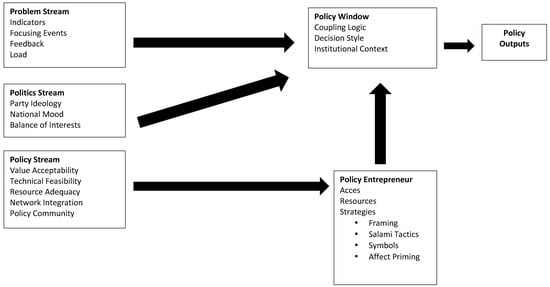The image is a detailed black-and-white flow diagram illustrating the process of policy formulation and implementation within an organization. The flowchart contains six black-outlined boxes connected by thick black arrows. In the first column from the left, there are three vertically stacked boxes labeled "Problem Stream," "Politics Stream," and "Policy Stream." The "Problem Stream" box includes terms like Indicators, Focusing Events, Feedback, and Load. The "Politics Stream" box features Party Ideology, National Mood, and Balance of Interests. The "Policy Stream" box lists Value Acceptability, Technical Feasibility, Resource Adequacy, Network Integration, and Policy Community.

Each of these three boxes points towards a central box labeled "Policy Window," which includes Coupling Logic, Decision Style, and Institutional Context. Below the "Policy Window" in the second column is a box labeled "Policy Entrepreneur," describing Access, Resources, and Strategies with a bullet list including Framing, Salami Tactics, Symbols, and Affect Priming. Finally, the "Policy Window" box points to the last box at the bottom labeled "Policy Outputs." This diagram visually represents the interactive and integrated approach to policy-making involving streams of problems, politics, and policy, culminating in eventual policy outputs.